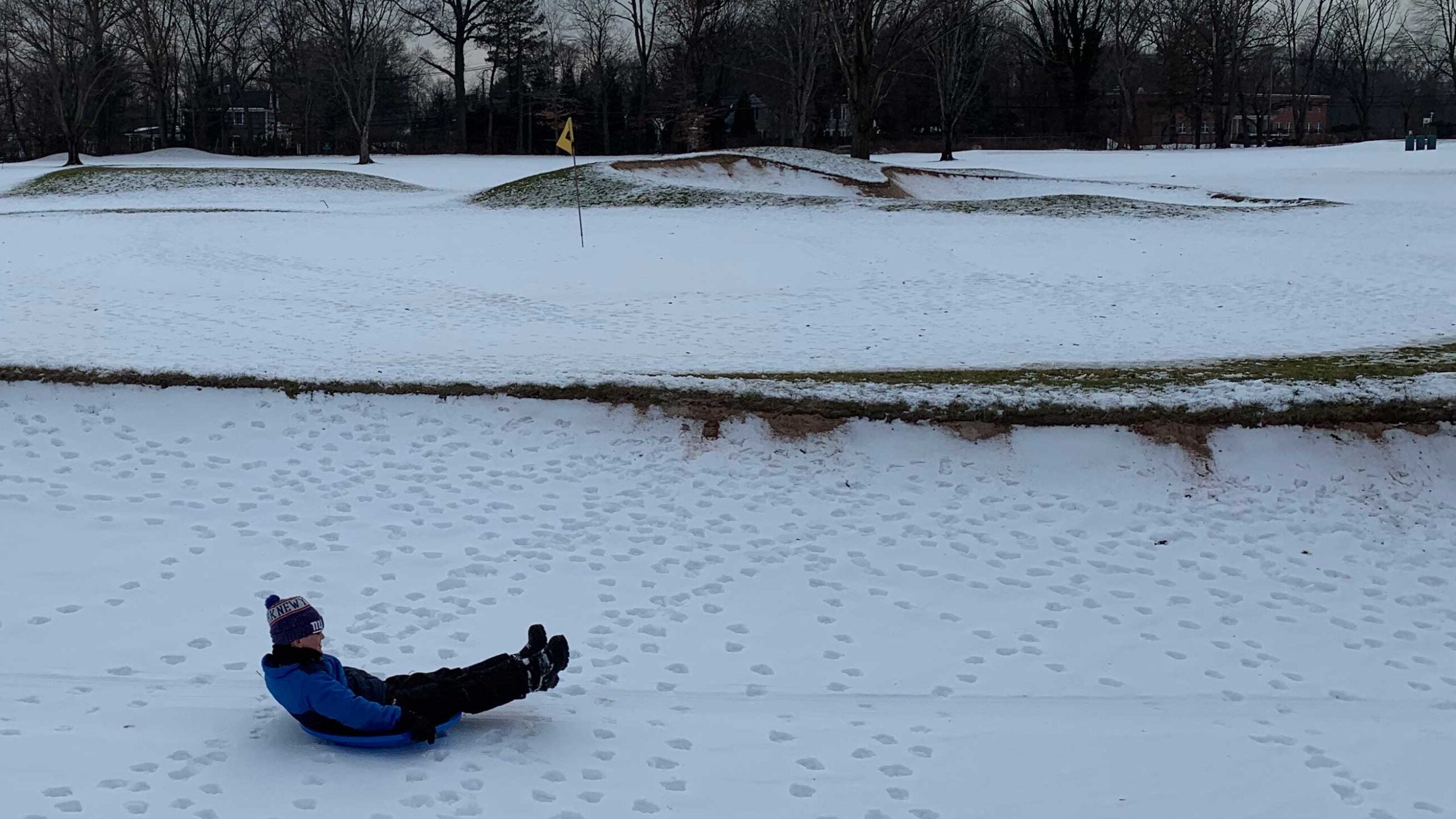The photograph captures a wintry scene, presumably on a golf course, with a landscape layout where the width is greater than the height. About 80% of the image is dominated by a snowy foreground, which is speckled with numerous small footprints suggesting recent activity. At the very top 20%, a row of dark, barren trees with visible branches punctuates the horizon under a likely overcast sky, adding to the bleakness of the scene.

In the lower left-hand corner of the image, a young boy, probably around ten years old, is depicted. He is bundled up in black pants, boots, a blue jacket, and a black beanie topped with a puff. The boy sits on a blue sled, a circular disk typically associated with casual snow play. His feet are pulled up, and his hands rest by his sides, suggesting a playful but static moment; there is no incline to facilitate actual sliding.

In the center of the photograph, a black line breaks the blanket of snow, possibly revealing the underlying land. Further back, additional hilly patches of snow can be seen, along with a flag with a yellow pennant, indicative of a golf green.

Despite the snowy cover, the overall scene is dark, likely due to poor lighting conditions or intentional camera settings, casting a somber tone over the landscape. The image is a striking representation of a winter day, where the elements of play and desolation intersect.